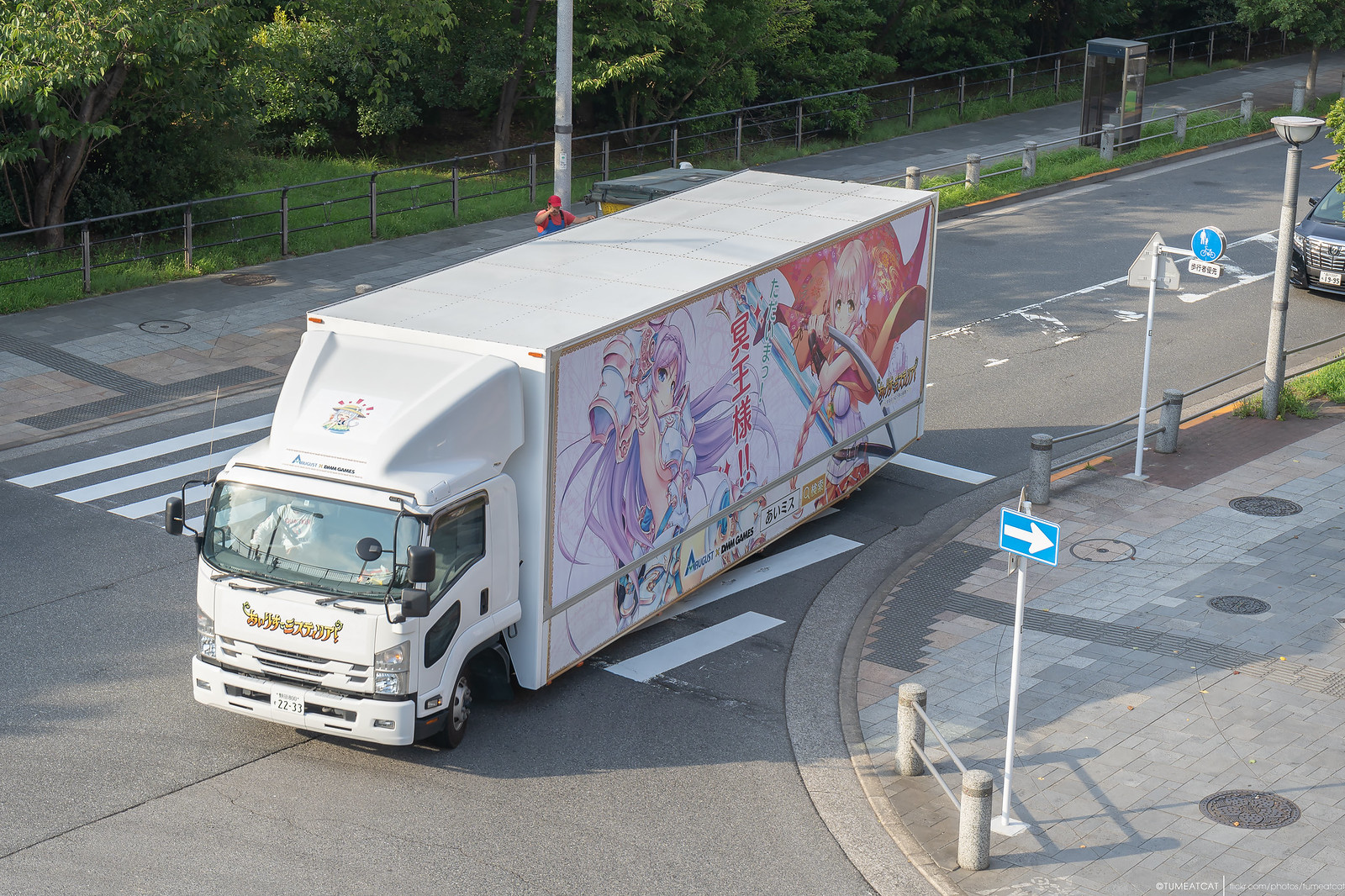On a two-lane roadway with a grayish asphalt surface, a large white panel truck drives down the street. The truck features an animated image on its left side, depicting two fairies with anime-style facial features. The left fairy has purple wings, purple hair, and a tan complexion, while the right one is adorned in rose and pink shades. The truck bears a yellow-orange name on its front. It appears to be turning left, guided by arrow poles indicating the direction on this highway. Following the truck at a distance is a small black car. In the background, a grassy area marks where the road ends. The truck is approximately 50 feet long, and the fine details of the animation are not fully visible due to the photo's distance.